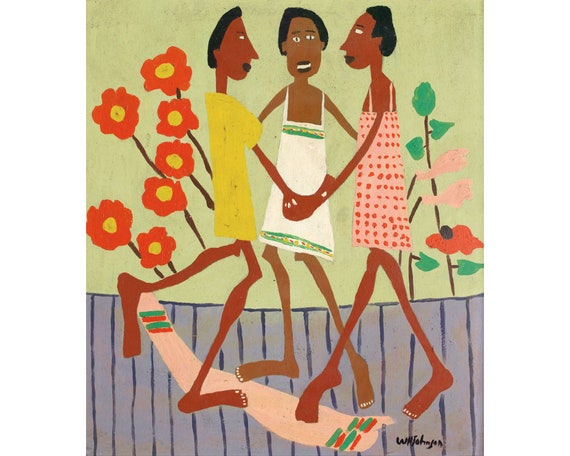This image features a hand-drawn, cartoon-like painting that depicts three young women dancing together in a circle, holding hands. They are all barefoot and have long legs with dark complexions ranging from brown to orangish skin tones. The woman in the center wears a white tank top dress with a green line around the top and bottom. To her left, one of the dancers is dressed in a yellow short-sleeve shirt, while the dancer on the right dons a pink dress adorned with red dots. Behind them is a lime green wall decorated with red and yellow flowers, to the left, and a green-leaved plant with pink flowers to the right. Above the women, the floor appears light purple with dark purple lines that signify the panels, and near their feet lies a garment or scarf, specifically a towel-like item with green and red stripes. The scene exudes a playful, joyous atmosphere, despite its minimalist, almost impressionist style. The artist’s signature is noted in the lower right corner but is too small and stylized to be legible.